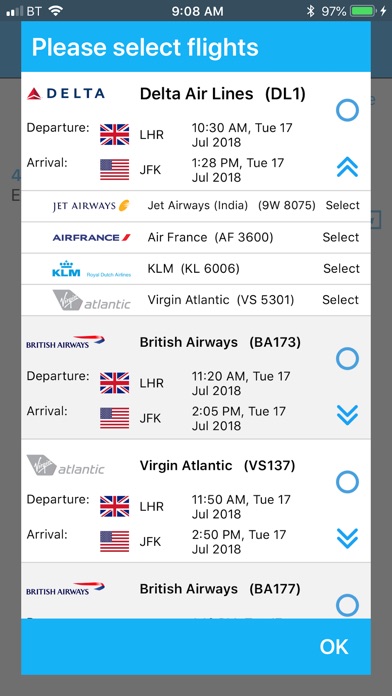This image displays a flight selection webpage. Centrally positioned, a list of airlines and respective flight details is shown, including Delta Airlines, Jet Airways, Air France, KLM, British Airways, and Virgin Atlantic. Next to each airline name are columns listing their departure and arrival times. Flags representing the UK and the United States are visible, symbolizing international travel options.

The top of the page features a distinctive red triangle adjacent to the word "Delta," indicating a highlight or special offer. A blue banner spans the top and bottom of the page, adding a cohesive design element. At the bottom of the page, a white-font "OK" button is prominently displayed on the blue banner, inviting users to confirm their flight selection.